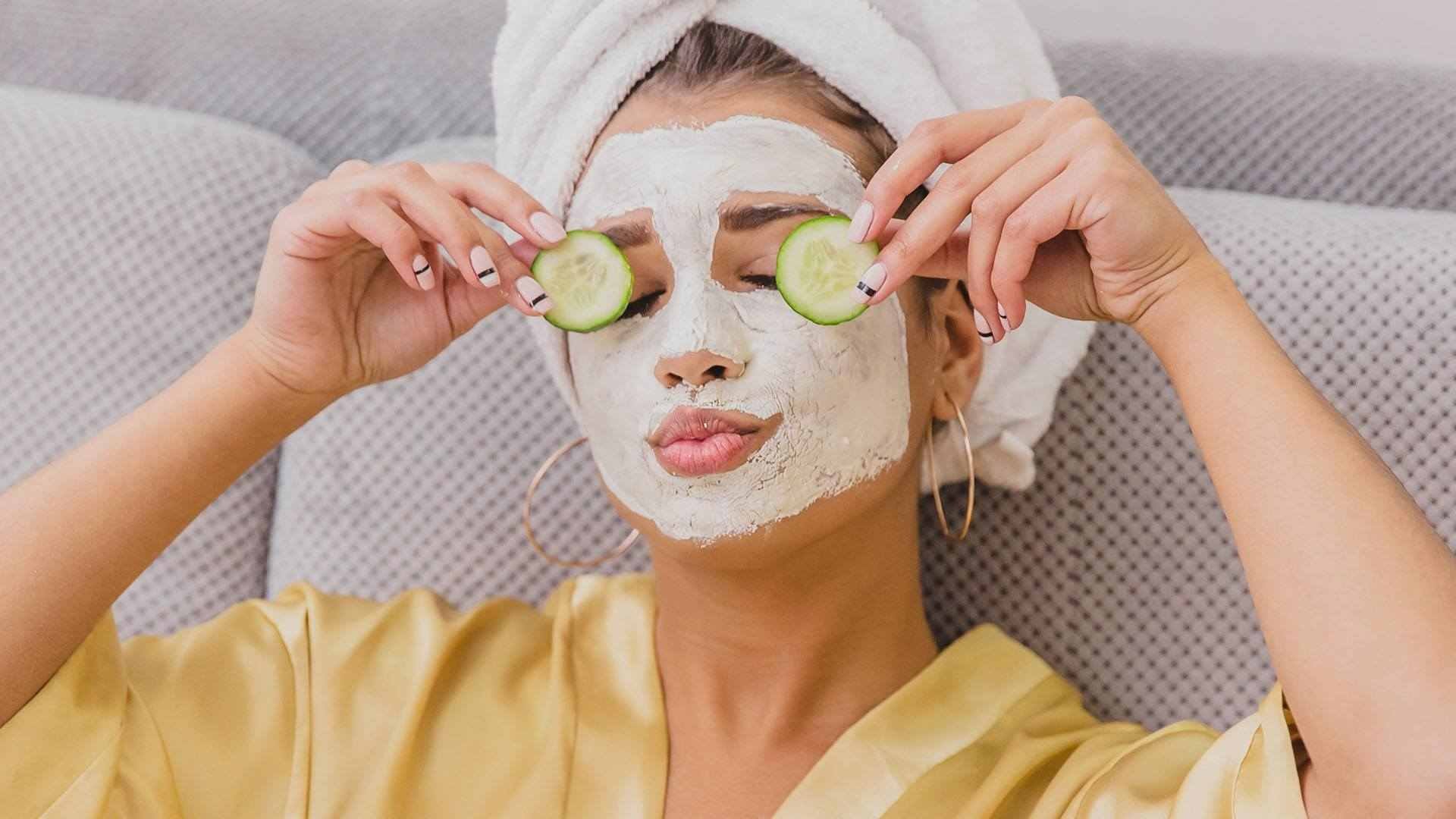This photograph captures a close-up moment of a Caucasian woman indulging in a facial. Dressed in a gold robe, she reclines against beige textured cushions, exuding calmness and relaxation. Her hair is neatly wrapped in a white towel turban, suggesting it may be freshly washed or protected. Her face is covered in a white mask that is beginning to dry, with only her lips, nose, and dark eyebrows visible. She is adorned with large, gold hoop earrings and has impeccably manicured nails painted white with black horizontal stripes. Her eyes are closed and her lips slightly pursed as she holds cucumber slices at the height of her eyes, preparing to place them on her eyelids. She looks serene and appears to be thoroughly enjoying this moment of self-care.